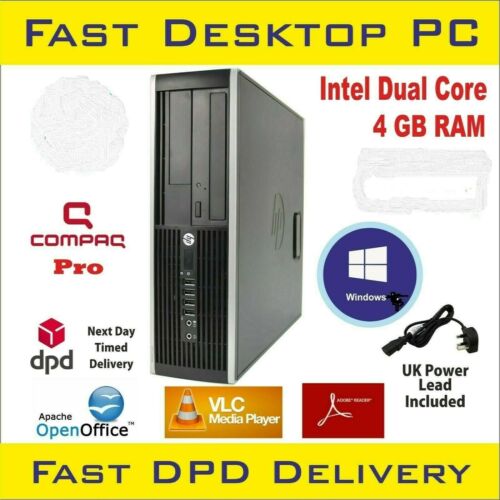This advertisement features a promotion for the "Compact Pro" fast desktop PC. It boasts impressive specifications, including an Intel Dual Core processor and 4GB of RAM, and is packaged with Apache Open Office software. The ad highlights the benefit of next-day delivery with a bold statement, "Fast DPD Delivery," displayed in a striking yellow and black font.

Prominently displayed is the Windows logo, set within a circular design where the outer ring is blue, transitioning to a purple inner circle. The word "Windows" is presented in white font, accompanied by a graphic representation of a four-pane window.

Additionally, the advertisement features the recognizable Adobe logo, which is red and white. For media enthusiasts, it also showcases the VLC Media Player logo, which is orange and rectangular, and includes an image of the iconic traffic cone, orange with white stripes.